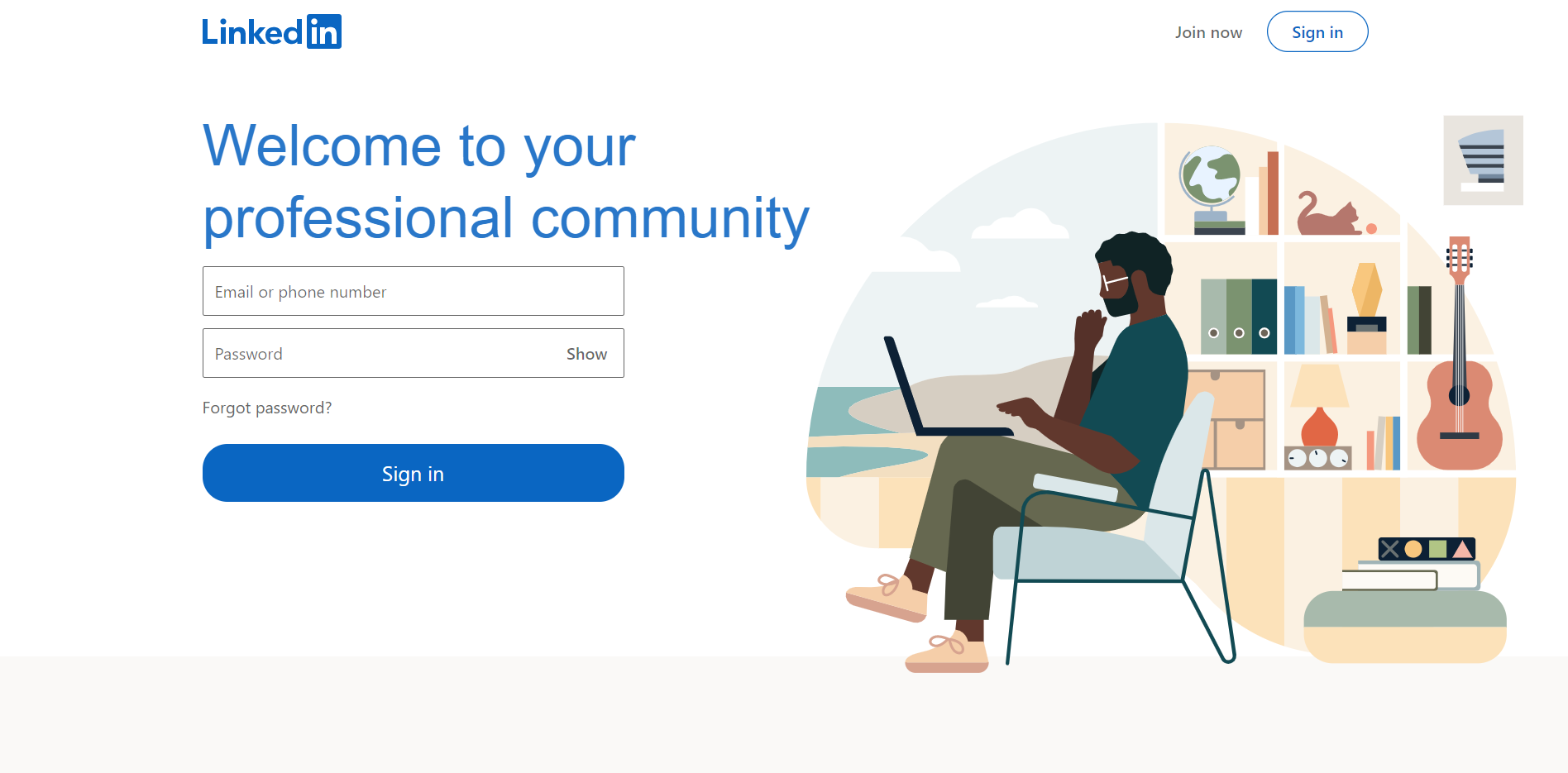This screenshot of a LinkedIn web page features a clean, white background. In the top left corner, the LinkedIn logo is prominently displayed with "LINKED" in blue text followed by "IN" in white text inside a blue square. In the top right corner, light gray text reading "JOIN NOW" is visible, adjacent to a white pill-shaped button outlined in light blue with "SIGN IN" in blue text at the center.

Below the logo, the main welcome message "WELCOME TO YOUR PROFESSIONAL COMMUNITY" is written in large blue text on the left side of the screen. Beneath this message are two text entry boxes with thin medium gray borders. The first box displays placeholder text "EMAIL OR PHONE NUMBER" in light gray, and the second box shows "PASSWORD" with a "SHOW" option in slightly smaller, darker text on the right side of the box. Below the PASSWORD field, aligned to the left, there is a "FORGOT PASSWORD?" link in light gray text. Directly below these fields, a blue pill-shaped button matching the width of the text boxes stands out with "SIGN IN" in white text.

On the right side of the screenshot, a simple, colorful illustration depicts a man seated in a chair. He wears green pants, a blue t-shirt, and pink shoes, complemented by black hair and white glasses. A black laptop rests on his lap. To his left, the illustration includes a rounded scene of a beach with a pale blue sky and white clouds, while to his right, there's another rounded scene showing a white bookshelf filled with books, a guitar, a globe, and other assorted objects.